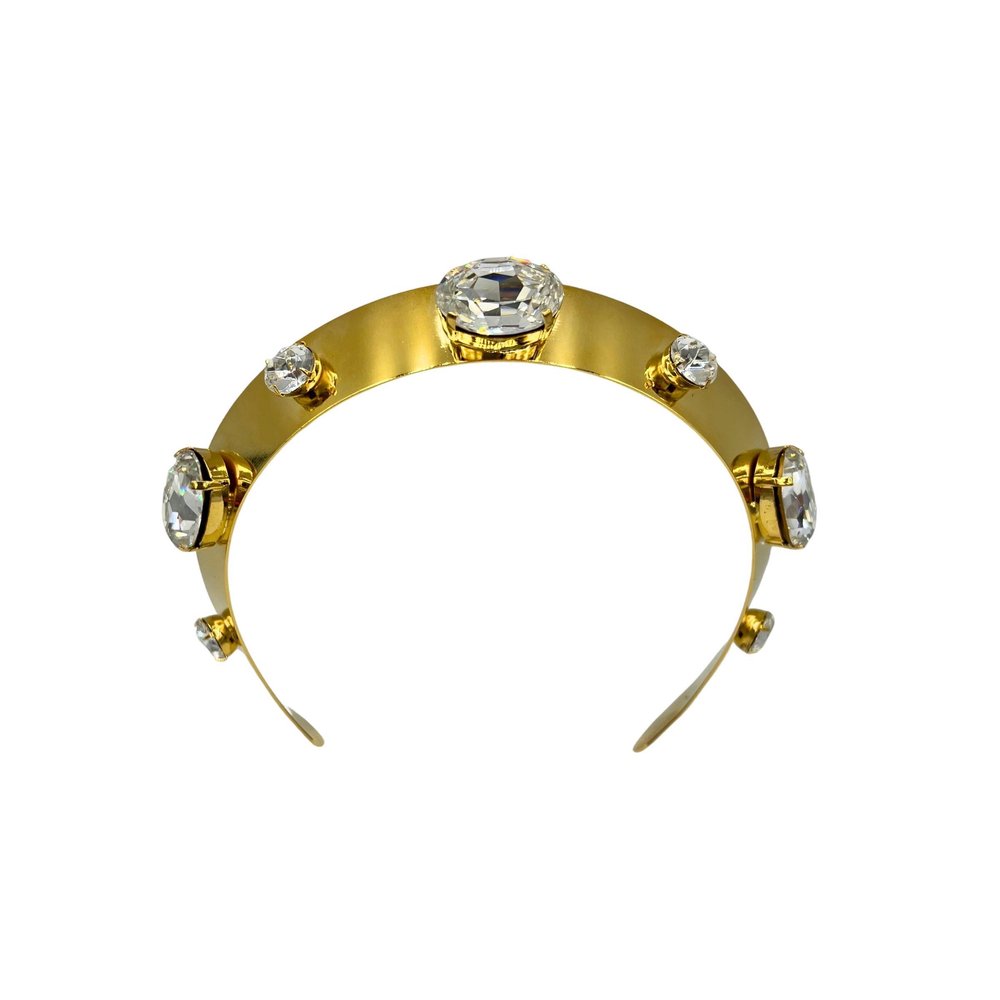A stunning piece of jewelry that appears to be a headband tiara, crafted from a golden or brass-looking material that could also be iron. The band is flat, smooth, and thick, with a flexible structure designed to curve around the forehead and head. It features a total of seven gems, alternately sized, beginning with a smaller one on the far left, followed by a larger one, and continuing in this alternating pattern. The central gem is the largest, drawing immediate attention with its silvery-white sparkle reminiscent of diamonds or rhinestones. The headband is set against a bright white background, highlighting its lustrous, shiny gold finish and intricate detailing in perfect focus, making it an exquisite adornment for a person.